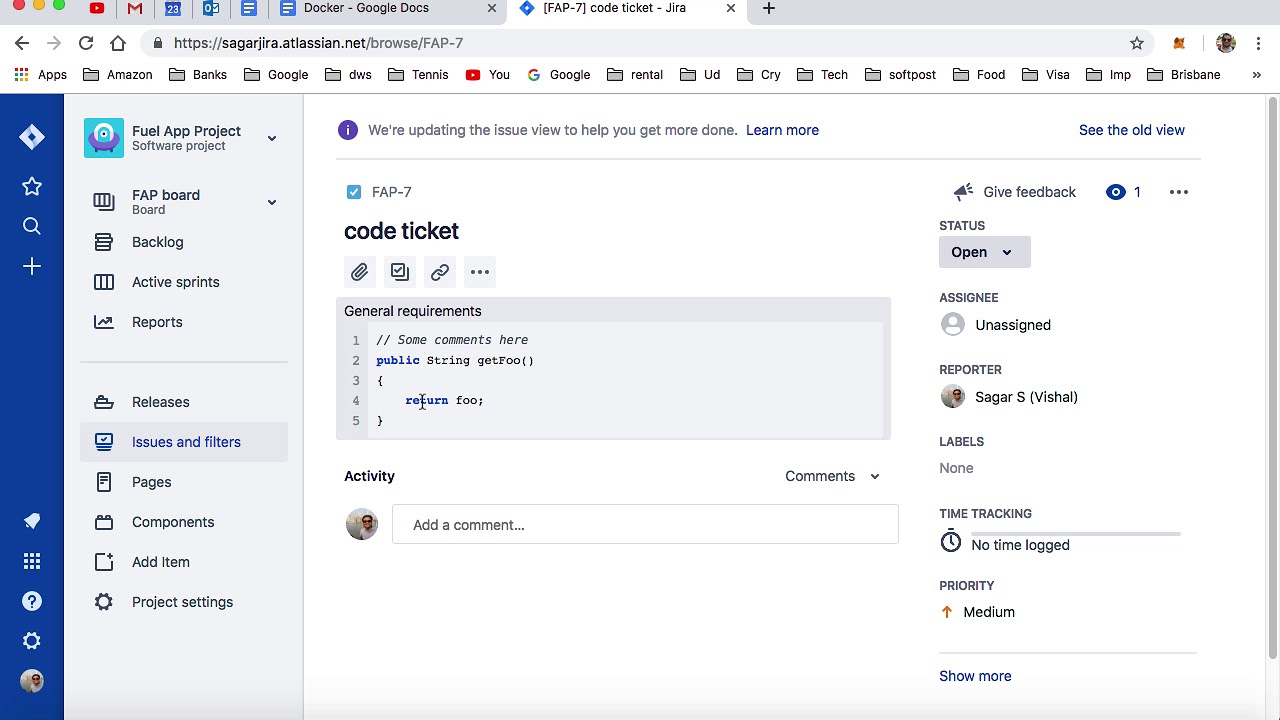**Detailed Caption:**

This image is a screenshot of a desktop browser page displaying a selected tab within a JIRA project management tool. At the top left corner of the browser window, the standard red, orange, and green buttons for closing, minimizing, and maximizing the window are visible. Several icons are arrayed, indicating accessible tabs or bookmarks, including YouTube, Gmail, Calendar, Outlook, two document icons, and a diamond icon labeled “FAP7 code ticket - JIRA,” which is the actively visible tab. Next to these, there is a plus icon allowing the user to add a new tab.

The typical browser navigation tools such as back, refresh, homepage, and the web address bar are present at the top, showing the URL: saga.adlesian.net/browse/FAP-7. Below the address bar, multiple bookmarks are noted.

The main content of the page is arranged with a blue left-hand vertical menu bar displaying various JIRA functionalities. From top to bottom, icons for JIRA, a star, search, add, notifications, main menu, help, settings, and the user’s profile picture are visible. Adjacent to this bar, a gray sidebar lists options such as "Fuel App Project," "Software Project," "FAP Board," "Board Backlog," "Active Sprints," "Reports," "Releases," "Issues and Filters" (the currently selected option), "Pages," "Components," "Add Item," and "Project Settings."

The central content area pertains to the "Issues and Filters" section with a highlighted JIRA issue (FAP-7). It begins with a notice stating that the issue view is being updated, offering links to learn more and view the old interface. The primary issue information includes:

- The issue ID: FAP-7
- The title: Code Ticket
- Icons for attachments, checkboxes, links, and additional options (three dots)
- A code block tagged "General Requirements" displaying a brief JavaScript function across five lines:
  ```
  // comments here
  public string getFoo() {
      return foo;
  }
  ```

On the right sidebar:

- A dropdown for "Status" marked as "Open"
- "Assignee": currently "Unassigned"
- "Reporter": "Sagar S.", with a note "(Vishal)"
- "Labels": "None"
- "Time Tracking": "No time logged"
- "Priority": marked "Medium"
- A "Show More" link offers additional details if needed.

Options such as adding comments, providing feedback, and viewing page actions are also available. The activity section notes one view and includes a dropdown to customize the display of comments.